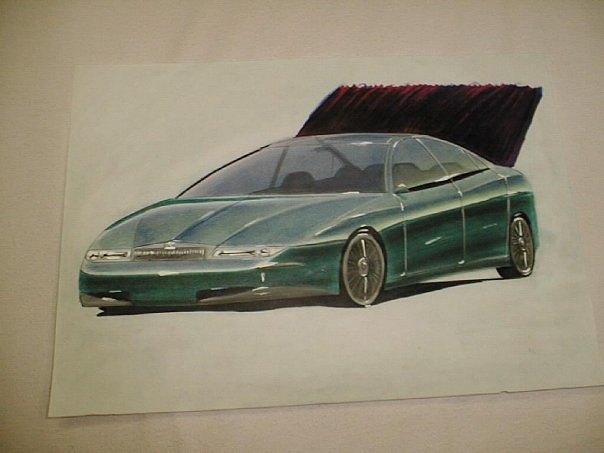This detailed drawing features a sleek sports car rendered in a dark greenish-blue hue. The car is strategically positioned to face the lower left corner of the white paper on which it is drawn. The background showcases a black road that gracefully extends from the trunk area towards the upper right, enhancing the sense of depth and motion in the artwork. A light source illuminates the car, casting reflections that highlight its polished surface. Only the two right-side tires are visible, adorned with elegant hubcaps that add a touch of sophistication. The artist has skillfully incorporated shadowing beneath the car, further emphasizing its three-dimensional form. The car’s windows are tinted, adding to its enigmatic allure. The drawing is set on an off-white table, providing a subtle contrast to the white paper and complementing the overall presentation.